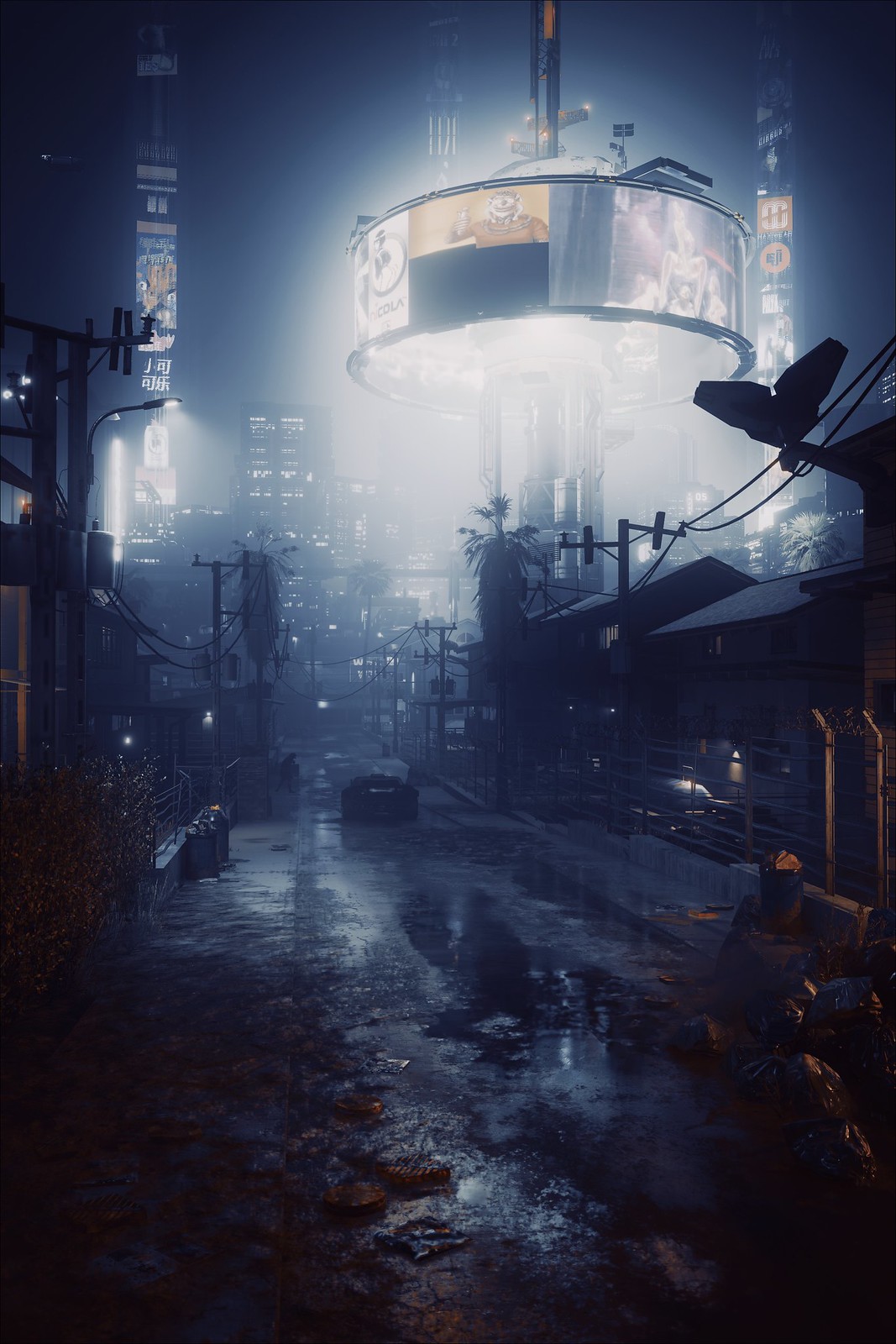A captivating night scene captures an urban street, likely a blend of real-world and digital elements, transformed by a recent rainfall. The road glistens with a reflective sheen from the water, enhancing the ambiance of the wet cityscape. Piles of trash are scattered along one side, adding a gritty, real-world touch to the environment. Alongside the street runs a low fencing, possibly topped with barbed wire, though the image's clarity makes it difficult to be certain. Strewn garbage litters the scene, contributing to the overall disheveled appearance.

Bright, vivid lights emanate from numerous advertisements and a few streetlights, casting an intense glow that drowns out the distant skyline and keeps the frame buzzing with energy. Silhouettes of tropical trees punctuate the urban environment, their forms barely discernible against the artificially lit backdrop. Residential buildings line the road, with power lines crisscrossing overhead and trailing off into the far distance, adding layers to the depth of the scene. Despite the overpowering lights, the late-night setting is unmistakable, the bright illuminations creating striking contrasts and casting long shadows throughout the damp, reflective street.